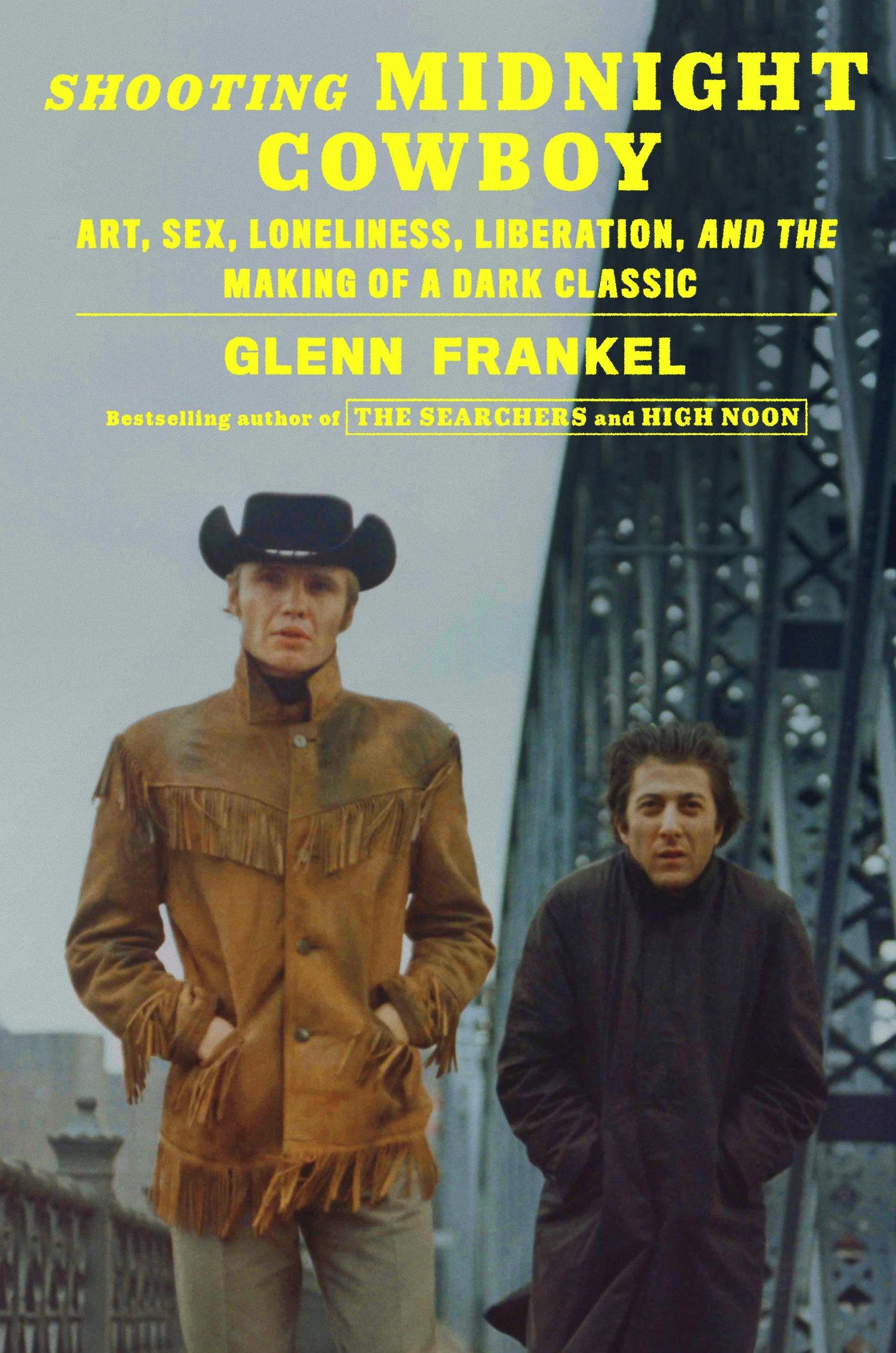The image appears to be a book cover for "Shooting Midnight Cowboy," featuring yellow text at the top of a vertical rectangle. In large capital letters, the title reads "Shooting Midnight Cowboy," followed by phrases in smaller yellow print: "Art, Sex, Loneliness, Liberation, and the Making of a Dark Classic." Below that, the author's name, Glenn Frankel, is highlighted, with a note that he is the best-selling author of "The Searchers" and "High Noon." The central image shows a scene from a movie, with two white men standing side by side, presumably actors John Voight and Dustin Hoffman. The taller man on the left wears a black cowboy hat, a brown leather jacket with fringe, and light-colored pants. He has blonde hair and no facial hair, with his hands in his pockets. The shorter man on the right, with dark hair, is dressed in a long black coat buttoned up to his chin, appearing hunched over as if cold, with his hands also in his pockets. Behind them, a city bridge with a gray, overcast sky sets the backdrop.